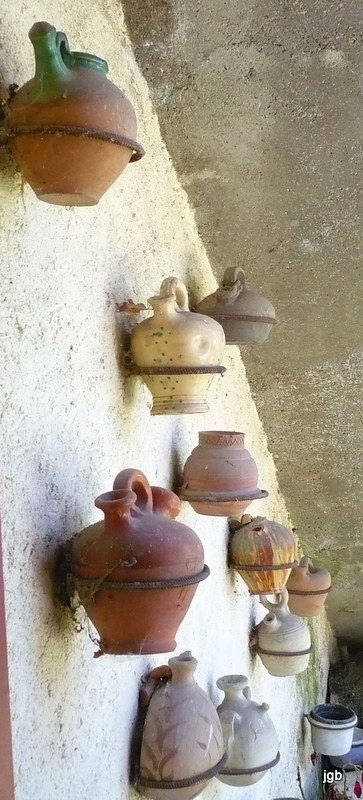The image, oriented vertically, depicts an ancient, rustic stucco wall with an aged, cracked concrete ceiling, likely in a museum setting reminiscent of Rome or Greece. Attached to the light brown, stone or plaster wall are metal loops holding a variety of amphoras and pottery jars. These amphoras, shaped like elongated beets with round tops tapering to narrow bottoms, are aligned in multiple rows. The collection includes eleven pots, featuring handles and spouts, with a range of colors from dark brick red to terracotta, with some displaying green upper portions. The pots, appearing handmade, vary in hues from gray to shades of red and tan. Notably, the upper left pot is terracotta with a green top and spout, and the lower left one is darker brick red with similar features. A plain white plant pot with a green interior is also visible at the bottom. The only marking on the image is "JGB" in the lower right corner.